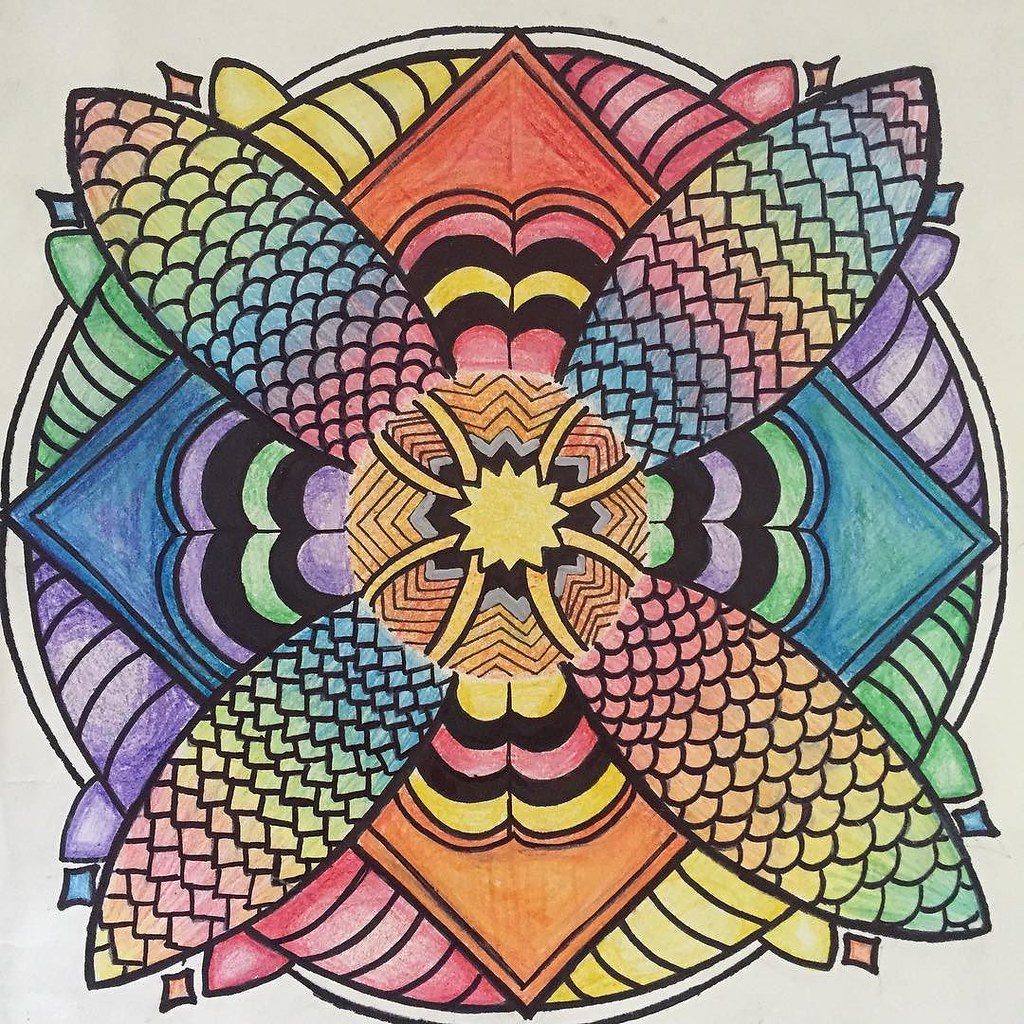The hand-drawn, colored-pencil artwork showcases a kaleidoscopic flower composed of intricate and symmetrical geometric patterns. At the center sits a star with numerous points, and it is enveloped by four petal-like shapes extending towards the corners of the image. These petals are adorned with a scaly pattern and shaded in vibrant hues of blue, green, yellow, pink, and orange. Surrounding the flower is a diamond-orientated square that appears as a rug-like design with intersecting lines and multi-colored sections. Concentric circles frame the square, adding depth to the composition. Additionally, a cloud-like bubble shape emerges under the petals, layered with double tram lines and imperfect concentric circles. Overall, the artwork bursts with an array of colors, including red, orange, mauve, black, and silver, all set against a light gray background. This piece, with its detailed symmetries and rich palette, has a mesmerizing and harmonious aesthetic.